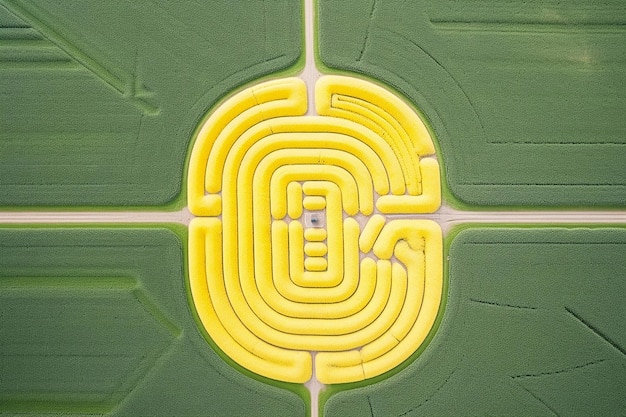The image appears to be a detailed aerial view of a vividly colored, artistic maze. The maze is split into four distinct sections, each surrounded by a lush green surface resembling grass or turf, much like a pool table. Radiating from the very center of the image are four white strips that resemble roads or walkways extending outward, intersecting at the yellow centerpiece. This centerpiece is an intricate, oval-shaped maze crafted from bright yellow materials that look like coiled balloons, play-doh, or elongated yellow clay tubes. The labyrinthine pattern in the middle evokes the appearance of a yellow brain. At the very heart of this yellow maze, there is a minute black object, difficult to identify but noticeable nonetheless. Whether an art installation or an imaginative architectural design, the image blends organic and artificial textures seamlessly, creating a captivating visual puzzle.